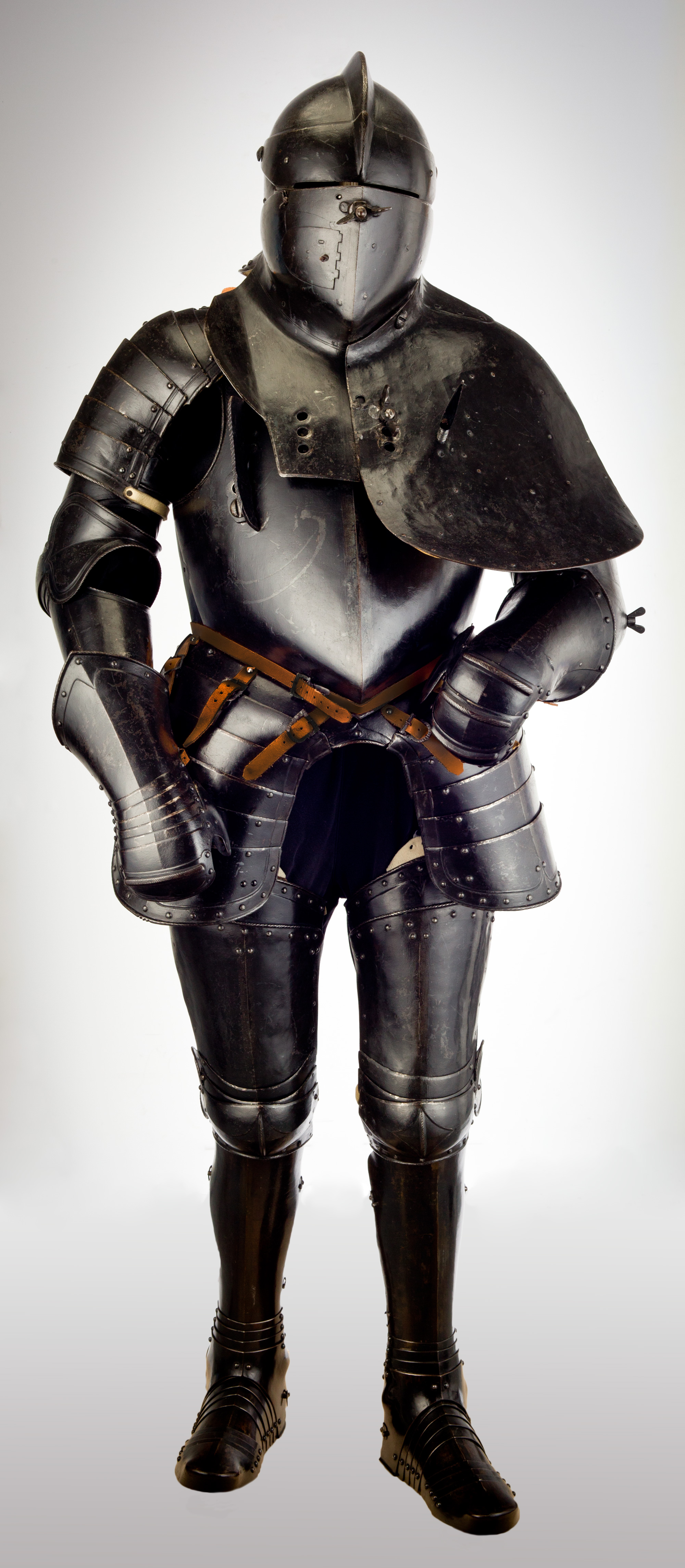This image showcases a professional, vertically-oriented photograph of an intricately detailed knight's armor, set against a light gray background punctuated by a central white light projection. The armor, composed of dark, gunmetal gray metal with a subtle shine, covers the figure from head to toe. Starting from the ground, the knight wears black boots that transition into silver-gray legging armor. The torso is predominantly light gray with orange accents around the waist area, resembling a belt. The left side of the torso features a protective metal plate to safeguard the heart, while the right shoulder and part of the arm are shielded by an extended piece of armor. The helmet, dark gray at the top and lighter at the bottom, is designed with narrow eye slits and small ventilation holes near the mouth, emphasizing the claustrophobic nature of wearing such protective gear. The ensemble is complemented by additional armor on the left side and a possibly ambiguous cape or skirt-like extension, contributing to an overall medieval aesthetic.